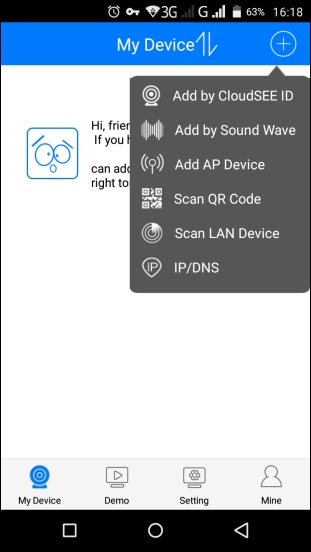A screenshot from a cell phone is prominently featured just left of the upper center. The status bar at the top shows various icons: an alarm clock, a key, a 3G signal indicator, four grayed-out vertical bars, a "G" symbol with four white vertical bars, and a vertical battery icon indicating 60% charge. The time displayed is 16:18. Directly below this, a blue header bar reads "My Device," flanked by an up-and-down arrow icon and a circular plus sign. 

On the right side near the top, a gray drop-down bubble contains several icons: beacons, waves, another beacon-like symbol, a QR code, a radar circle, and an IP icon inside a badge. To the right of these icons, there are headers labeled "Add by Cloud SEE ID," "Add by Sound Wave," "Add AP Device," "Scan QR Code," "Scan LAN Device," and "IP/DNS."

Below these headers, a thin square with rounded corners features a cartoon face and the greeting, "Hi friend," followed by partially obscured text due to the drop-down menu overlay. The text appears to instruct on adding a device but remains unreadable in parts.

At the bottom of the screen, four options are listed: "My Device" (highlighted in blue), "Demo," "Settings," and "Mine." The navigation bar at the very bottom features white buttons on a black background.